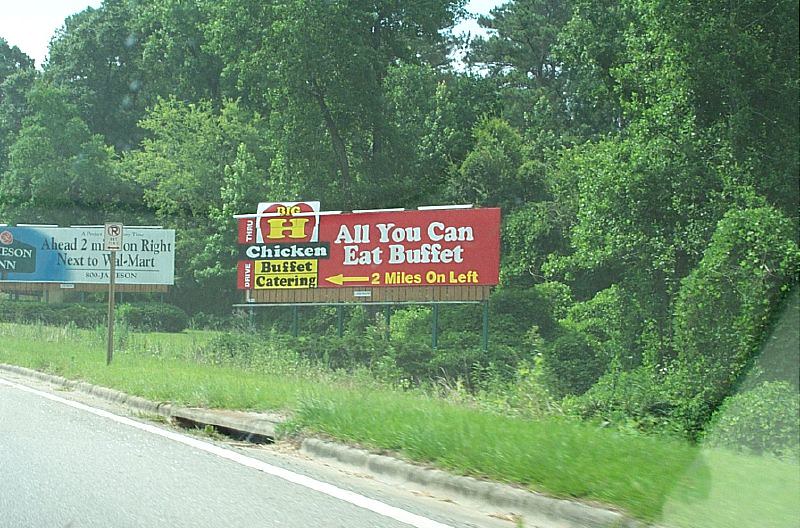The photograph captures a scene viewed from inside a car, likely taken from the passenger seat. Dominating the foreground is a large billboard advertising an "All You Can Eat Buffet" located two miles on the left. The billboard promotes the "Big H Chicken Buffet Catering" and mentions a drive-thru option. The locale appears to be rural, characterized by large trees and tall grass surrounding the area.

In the background, another billboard is faintly visible; though less legible, it seems to advertise something akin to "Jameson Inn," located two miles ahead on the right, next to a Walmart. A no parking sign is positioned near the side of the road, and a rain gutter is also visible, suggesting the presence of a well-maintained infrastructure.